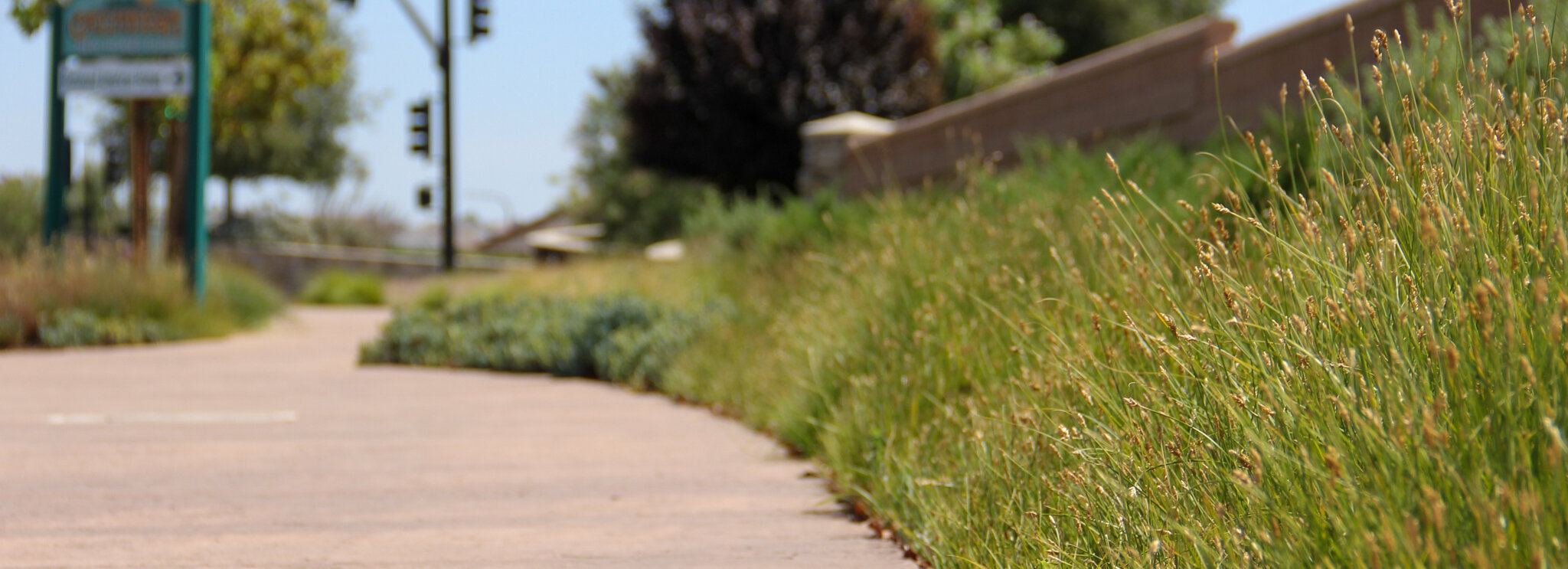A detailed and structured caption for the image could be:

"Displayed is an urban scene featuring a light grey cement sidewalk with subtle shades of reddish-brown. Flanking the sidewalk to the right is a verdant expanse of tall green grass, culminating in a layered brown stone fence that gradually ascends as it stretches further into the background and lowers closer to the viewer. Beyond the fence, a striking grove of mixed red and green trees adds depth and color to the scene. To the left of the sidewalk stands a black traffic light pole, hosting two signal lights; one faces left and the other, positioned higher, faces right. The sky above is a clear, vibrant blue. On the left side of the image, another green tree is visible, and beneath it, there are two green poles holding signs. The upper sign is green with orange lettering, and directly beneath it, a white sign with black lettering. Additional tall green grass grows around the base of these poles. A faded white line is faintly visible on the sidewalk towards the left-center of the image."